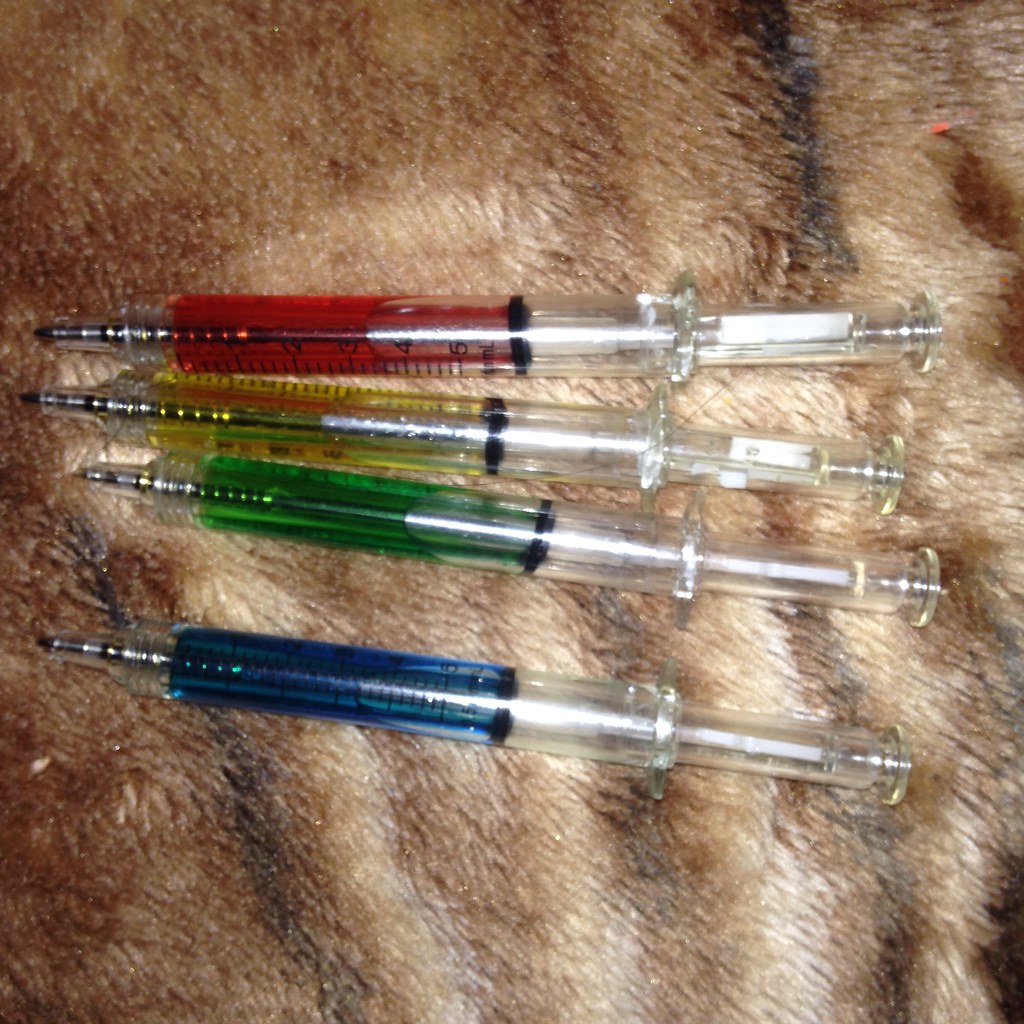The color photograph shows an overhead view of four hypodermic needles arranged horizontally, side-by-side, almost spanning the entire width of the image. The needles rest on a textured, brown rug with lighter beige tones and black vertical stripes, creating a multi-colored, furry backdrop. Each needle has a translucent plastic body and is approximately two-thirds full with liquids of different colors—red at the top, followed by yellow, green, and blue at the bottom. The needles are oriented with their points, covered by plastic caps, to the left and the plungers on the right. The lighting in the photograph highlights parts of the needles and adds a sense of depth to the image.